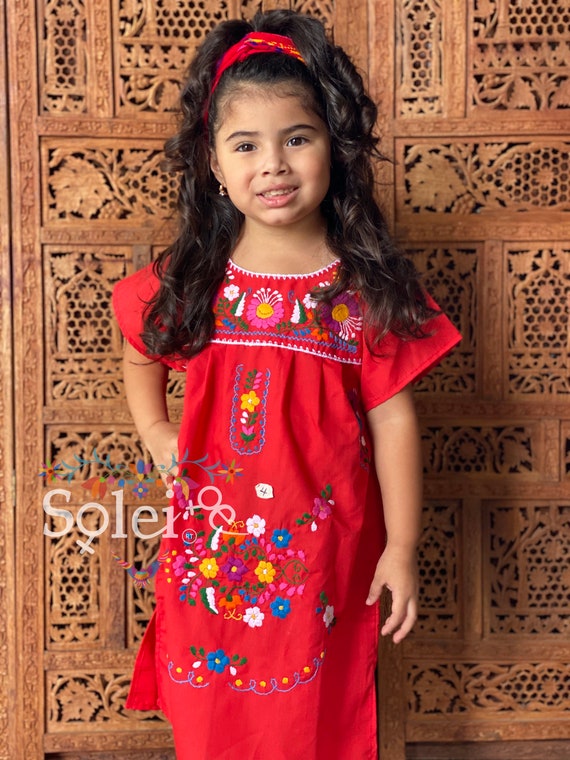The photograph features a young girl with long, wavy black hair, partially held back by a red headband. She is dressed in a vibrant red dress adorned with a variety of colorful floral patterns in yellow, pink, blue, and green. The girl's skin tone suggests she may be of Asian or South Asian descent, and she sports a pair of earrings. She stands confidently, with one hand on her hip and the other resting by her side, looking straight into the camera with a partial smile. The background appears to be an ornately designed wooden panel or door, decorated with a combination of honeycomb and plant motifs, including leaves and flowers, arranged in rectangular sections. The scene is further detailed by semi-transparent white text on the left side of the image that reads "Soleil," potentially a name or a brand watermark. The photograph cuts off just below the girl's knees, providing a focused yet detailed view of her and her attire.